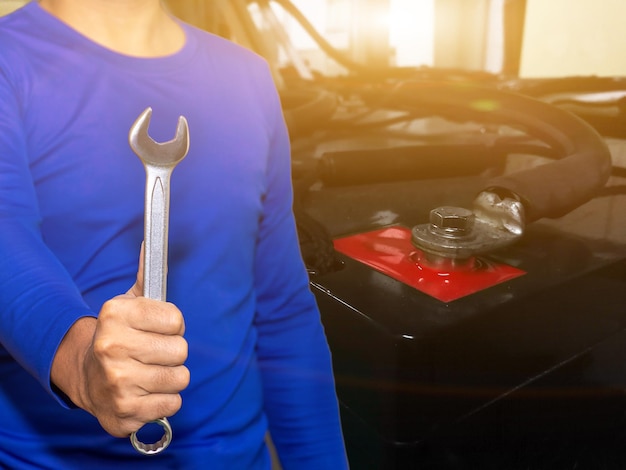In this color photograph, we see a person's torso clad in a bright blue long-sleeve t-shirt. Their face is not visible, as the image is cropped from their neck down to their waist. They are gripping a wrench tightly in their right hand, which is extended towards the camera. The wrench has an open end and a socket end, indicating it is a versatile tool. Standing next to them, on the right side of the image, is a large, intricate machine. This machine resembles an oversized car engine or possibly an electrical unit, with a big bolt and numerous wires disappearing into the background. The machine's components are predominantly black with a bit of red, suggesting insulation material or a connector plate. The setting appears to be a garage bathed in bright sunlight, making the mechanical details stand out in sharp relief.